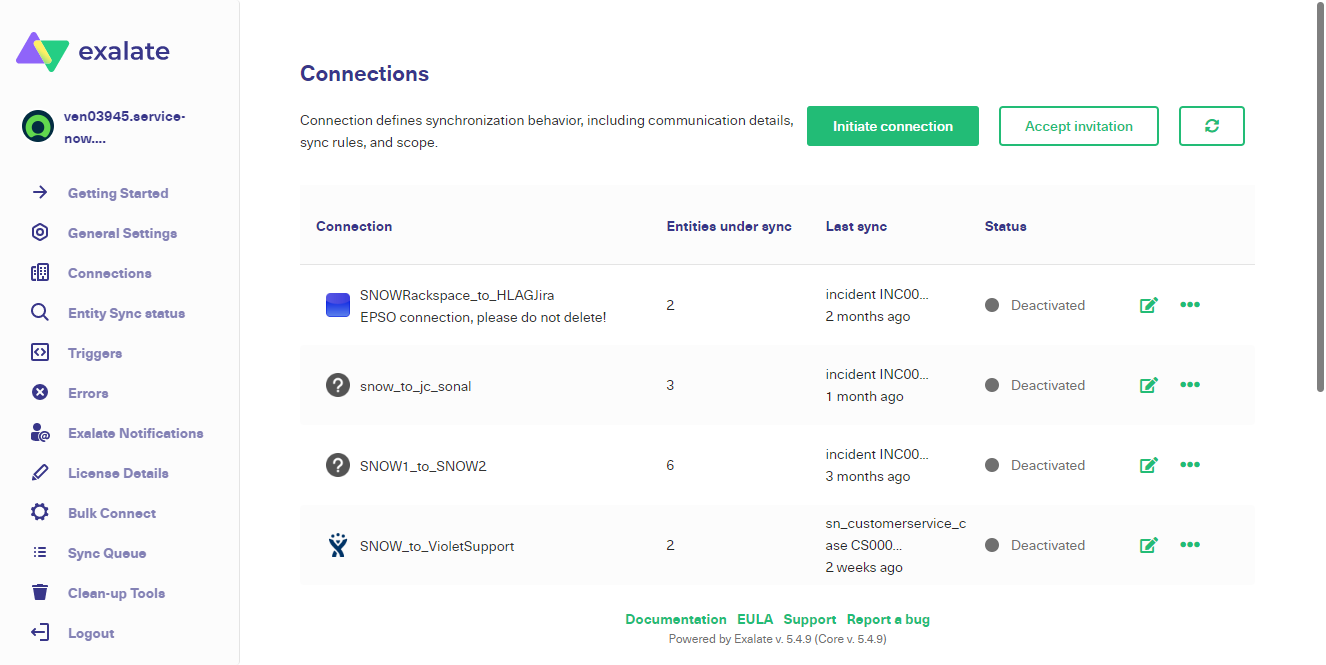This image showcases a screenshot from Exalate, a synchronization tool. The Exalate logo, prominently displayed at the top, features a distinct emblem composed of a purple triangle partially overlapped by an upside-down green triangle, with a yellow stripe in the upper left corner of the green triangle.

On the left side of the screen, under the Exalate heading, there is a navigation menu. This menu is identifiable by a green-circled icon depicting a small head, suggesting user settings or information. The options listed in this column include: Getting Started, General Settings, Connections, Entry Sync, Triggers, Errors, Exalate Notifications, License Details, Bulk Connect, Sync Cues, Cleanup Tools, and Logout.

To the right of the navigation pane, in a main content area formatted with five columns, the section is titled "Connections." This section outlines the purpose of a connection within Exalate, explaining that a connection defines synchronization behavior by including communication details, sync rules, and scope.